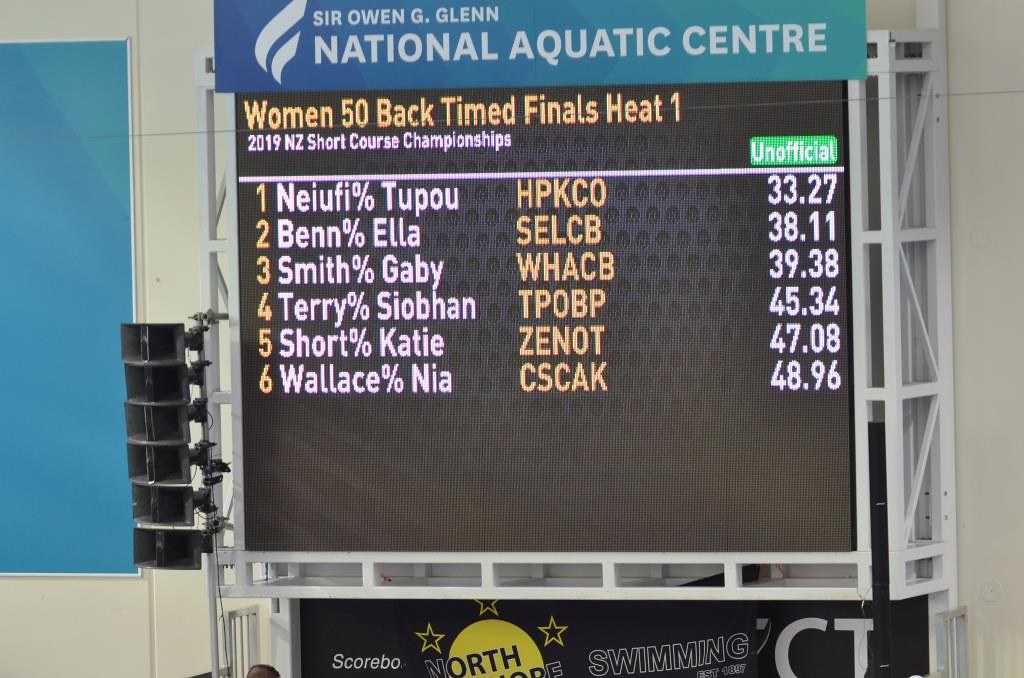This photograph captures a detailed view of the scoreboard at the Sir Owen G. Glenn National Aquatic Center during the 2019 NZ Short Course Championships. The image is wider than it is tall, depicting a sophisticated black metallic display board mounted on a white tiled wall. The scoreboard is held up by a metallic frame with speakers attached to it.

At the very top of the scoreboard, a prominent banner transitions from deep blue on the left to a lighter blue-green on the right, bearing the text "Sir Owen G. Glenn National Aquatic Center" in gray print. Just below this banner, another black banner displays "Scorbo Swimming" in white print, though the full text appears incomplete.

The main part of the scoreboard begins with the event title in yellow or orange text: "Women 50 Back Timed Finals Heat One." Beneath this, in smaller white print, is the text, "2019 NZ Short Course Championships." A horizontal white line demarcates the start of the results. The scoreboard lists competitors in six rows, starting with the placement number (1 to 6) in orange, followed by the swimmer's name in white. Each entry provides detailed information including an identifier for the swimmer’s team in orange and their unofficial race time in white.

1. **Newfie Tapu (HPKCO)** - 33.27 seconds
2. **Benn Ella (SELCB)** - 38.11 seconds
3. **Smith Gabby (WHACB)** - 39.38 seconds
4. **Terry Siobhan (TPOBP)** - 45.34 seconds
5. **Short Katie (ZENOT)** - 47.08 seconds
6. **Wallace Nia (CSCAK)** - 48.96 seconds

Each swimmer’s team or organization is denoted with letters and symbols, and the times listed are marked as unofficial. These diverse pieces of information concisely capture the competitive standings and individual details of the swimmers, making the scoreboard an integral part of the swim meet's documentation.